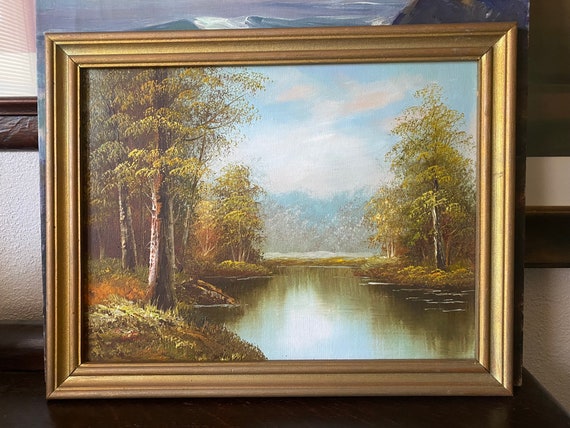The image showcases a painting housed in a fairly thick, ornate golden frame, measuring approximately 12 inches by 16 inches. This framed artwork sits atop a dark, shiny wooden table, with a portion of a white textured wall and a brown ledge visible both above and below it. Behind the framed painting is another piece of unframed artwork, partially visible with hints of blue emerging from its top. 

The painting itself is a natural landscape, depicting a tranquil, small body of water—possibly a pond or swamp—set amidst a verdant, wooded area. The water reflects the surrounding trees and the blue sky above, complete with scattered white clouds. The banks of this water body are lined with trees, featuring a mix of green and transitioning fall colors, suggesting the onset of autumn. The trees, with their full array of leaves, flank the scene on the left and right, contributing to the darker green hues reflected in the water. The background of the painting extends into the horizon, revealing more trees against the cloudy sky. The photograph capturing this framed painting hints at it possibly being up for sale, adding an element of commerce to the scene.